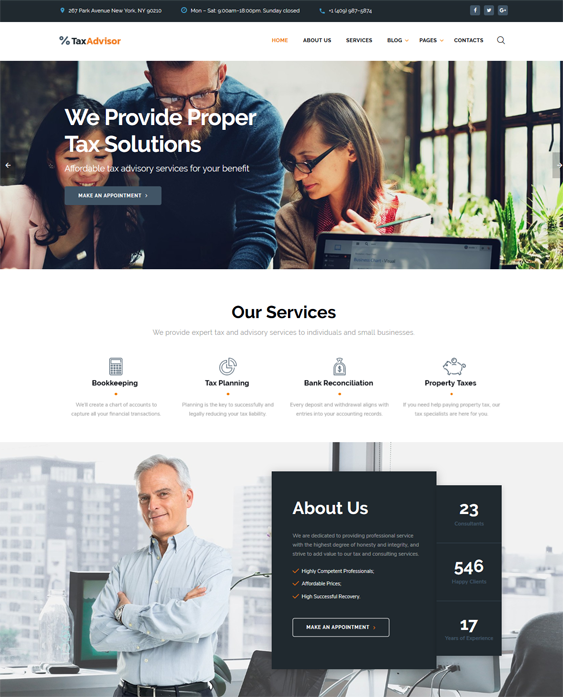This image appears to be a screenshot from a professional website with a focus on tax and advisory services. The image features a distinct layout with multiple sections:

At the top, a black navigation bar stretches across the width of the image, roughly an inch thick. On the left-hand side of this bar is a blue icon, followed by some white text. Adjacent to this is a blue circle containing additional white text that is difficult to discern. Next, there is a blue icon resembling the handset of an old-fashioned telephone, followed by more white text. On the right side of the bar, three gray boxes house white icons that are indeterminate.

Below the navigation bar, the background transitions to white. In the top-left corner, the text "%taxadvisor" is displayed, with "tax" in black and "advisor" in orange. To the right of this, several navigation links are listed: "Home" in orange, "About Us" in black, "Services" in black, "Blog" in black, "Pages" in black, "Contacts" in black, and an icon that looks like a black spyglass.

A photograph is situated beneath this section. On the left, an Asian woman with black hair, dressed in a pink coat, is visible. Next to her, a Caucasian man with black-rimmed glasses, a blue button-up shirt, and a beard is seated. To his right, a woman with shoulder-length brown hair and black glasses looks to the left. All individuals are positioned in front of a computer, seemingly engaged in work.

Below the photograph, the text "Our Services" is prominently displayed in bold black font. Underneath, in gray text, it reads, "We provide expert tax and advisory services to individuals and small businesses." Following this, several icons and descriptions of services are listed horizontally:
- A calculator icon with the label "Bookkeeping."
- A black symbol with the label "Tax Planning."
- A money bag icon with the label "Bank Reconciliation."
- A piggy bank icon with the label "Property Taxes."

At the bottom, a picture of an elderly man with gray hair, wearing a blue button-up shirt, appears. Next to him, a black bar contains white text that reads "About Us."

Overall, the image depicts a professional, well-organized website, focused on providing a range of tax and advisory services.